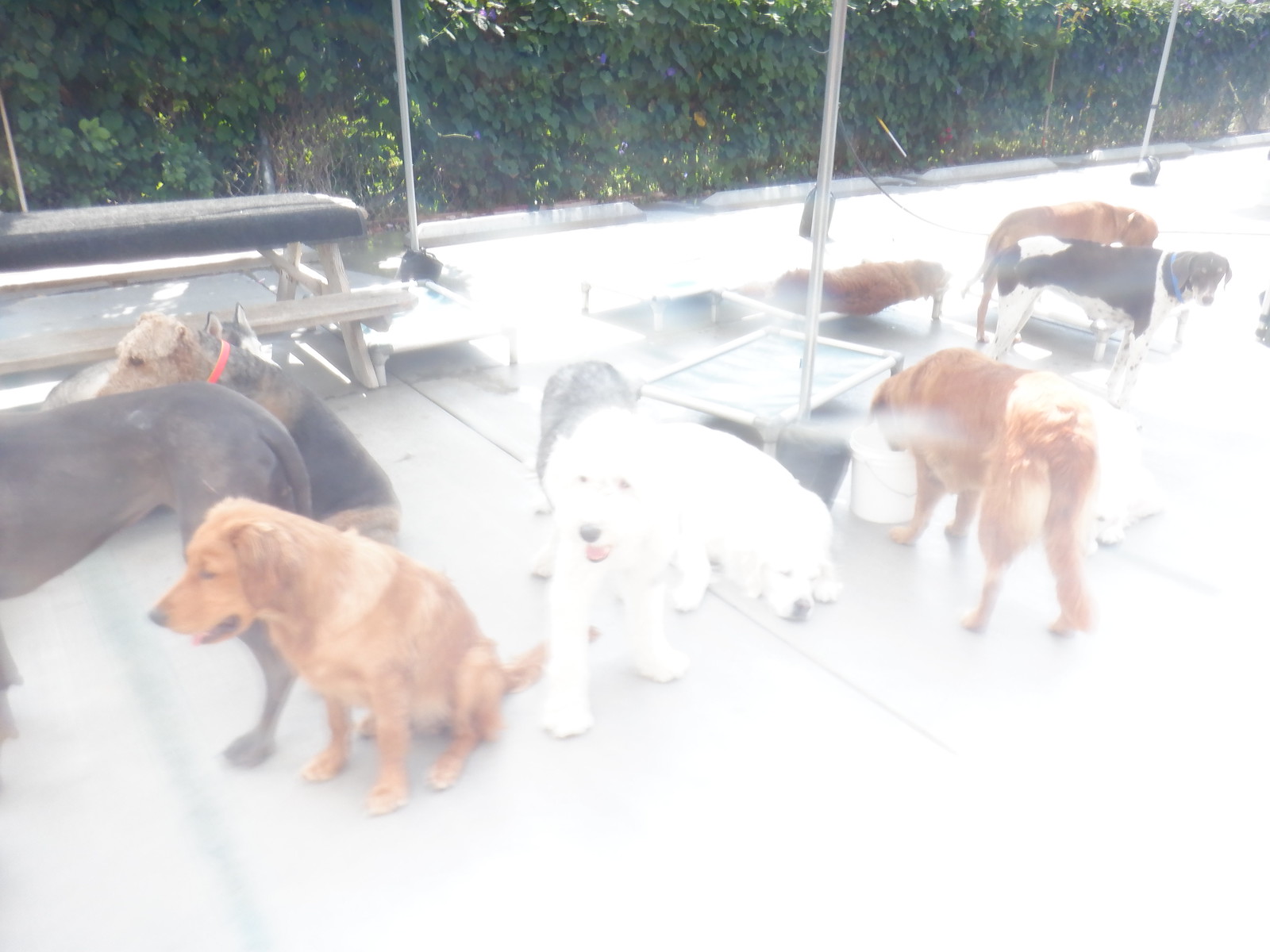This outdoor photo, despite its poor quality with smudges and blur, captures a vivid scene of ten dogs in a fenced area. A green hedge forms the backdrop, partially obscured by the brightness that washes over the image. The ground appears to be a concrete or white tile patio. To the left, a light brown park bench with a black cushion is visible, along with several raised dog beds and picnic tables.

The dogs are varied in breed, size, and color. Central in the image is a large, white Great Pyrenees, laying down. Next to it, a smaller sheepdog and two orangish Golden Retrievers are visible. One Golden Retriever is sitting, while the other is drinking from a bucket. Another large dog, possibly a Great Dane, stands nearby, partially cut out of the frame. A dark brown dog with white legs and underbelly stands to the back right, while a smaller, dark brown dog with a light brown face and red collar sits behind it. Further back is a dog that looks part beagle with a blue collar and another that seems to be a dachshund. One dog appears to be a Schnauzer with a red collar, and a terrier with a black back and tan head can be seen behind it. An orange poodle is lying down on one of the raised dog beds. The dogs are spread throughout the image, creating a lively and somewhat chaotic scene despite the photo's clarity issues.